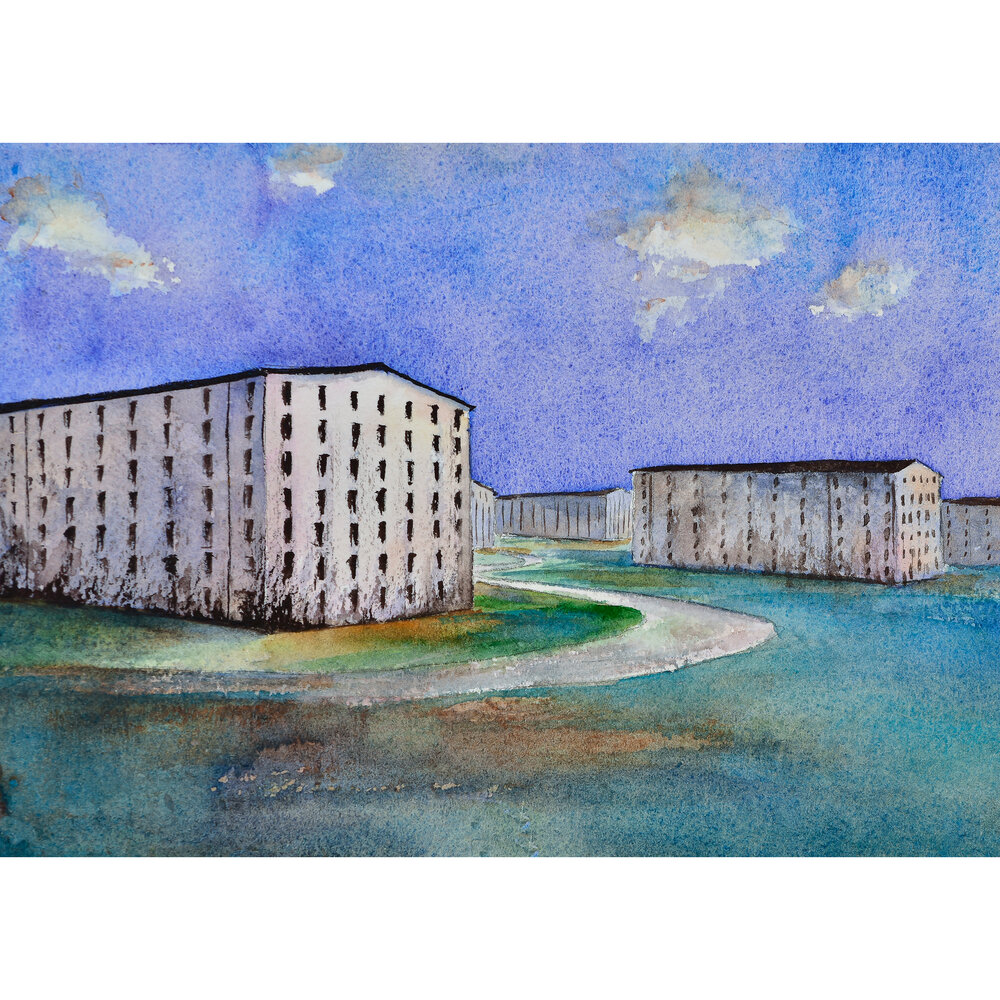This hand-painted watercolor image depicts a cluster of several large, rectangular, multi-story buildings, each with many black, grid-aligned windows on their white facades and narrow, gently sloped black roofs. The buildings are arranged either fully or partially in view, some side-by-side, and some appearing more prominent than others. A mottled sky with shades of blue and purple, speckled with light clouds creates a striking backdrop. The foreground features a mix of brown, green, and blue brushstrokes that suggest a watery expanse or shoreline, alongside patches of gray indicating a curvy path or road winding through the scene. The overall style of the painting is rudimentary and hand-crafted, adding a raw, interpretive essence to this landscape.